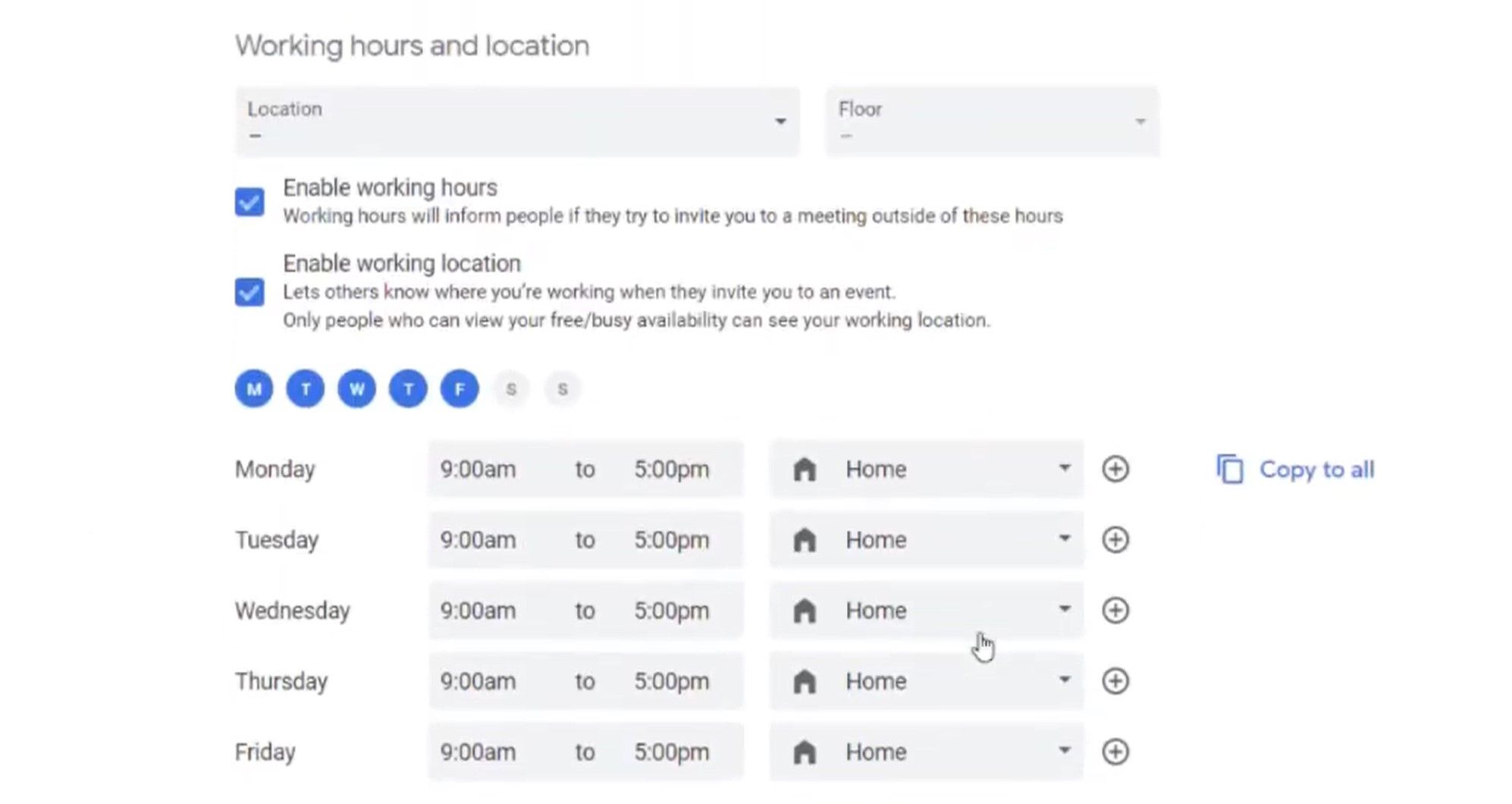The image displays a user interface designed for setting work hours and locations, likely from a calendar or scheduling application. At the top, the section is titled "Working Hours and Location." There is a dropdown menu labeled "Location" currently displaying a placeholder, alongside another dropdown for selecting the floor, also showing a placeholder indicated by a dash. Below, two checkboxes are present: one labeled "Enable Working Hours," which is checked, accompanied by text explaining that "Working Hours will inform people if they try to invite you to a meeting outside of these hours." The second checkbox, "Enable Working Location," is also checked, with text stating, "Let others know where you are working when they invite you to an event. Only people who can view your free/busy availability can see your working location."

The interface allows users to select workdays, with Monday through Friday highlighted and Saturday and Sunday left blank. Each weekday, Monday through Friday, shares the same schedule: starting at 9 AM and ending at 5 PM, with the location set to "Home," identified by a house icon. A plus sign is available for adding more time slots. Additionally, "Copy all" links are provided to replicate the settings across all selected days, streamlining the process of defining work hours and locations.

Overall, the layout offers clear instructions and user-friendly controls, making it straightforward for users to specify their availability and working locations for each day of the week.